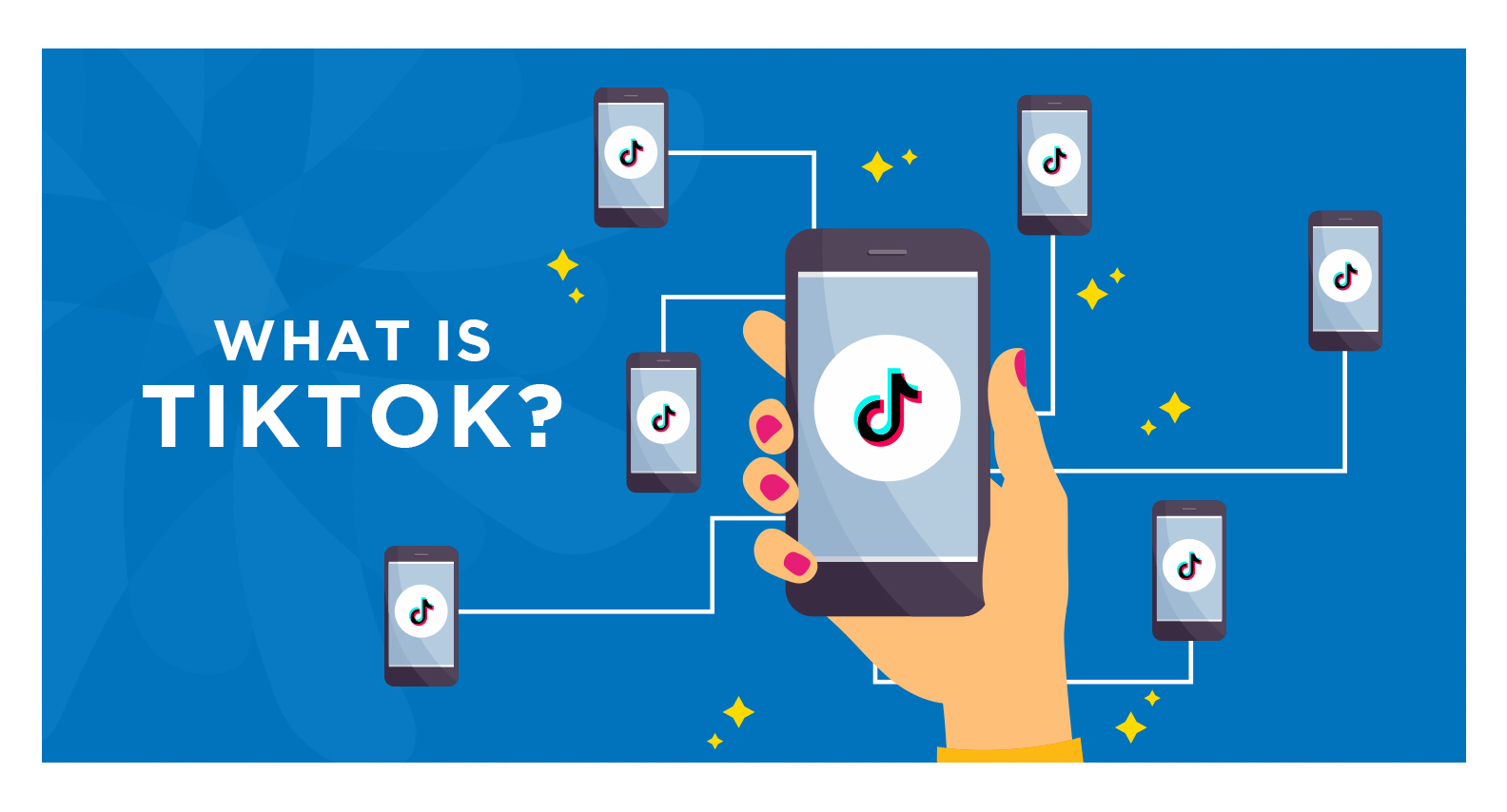This image features a solid blue background that gradually transitions into a mix of darker and lighter blue tones on the right side, creating a subtle, fanned effect. Over this background, in prominent white text, the question "What is TikTok?" is displayed. Additionally, the image includes a cartoon-style animation of a right hand, palm facing forward, holding a cell phone. The hand is adorned with pink nail polish and has a yellow cuff at the wrist, suggesting the edge of a piece of clothing.

The cell phone held by the hand has a black outline and a gray screen, prominently displaying the TikTok logo within a white circle. From this central device, six white lines radiate outward, each leading to smaller, identical cell phone icons also featuring the TikTok logo. Scattered randomly throughout the image are yellow stars, adding a playful touch to the overall design.